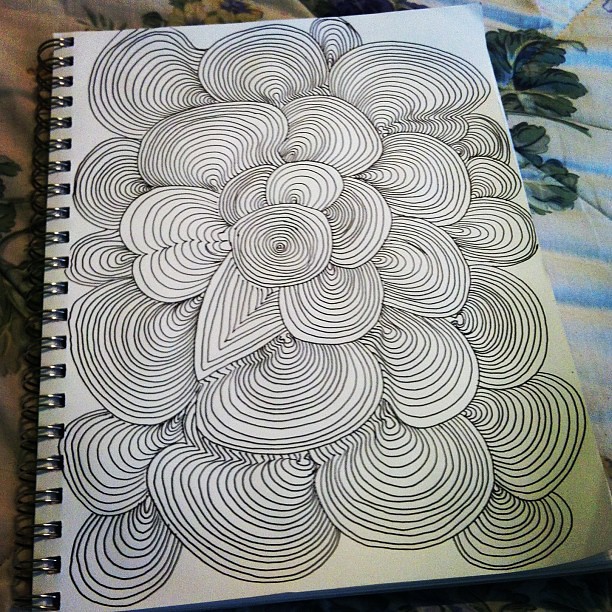A square image displays a notebook resting on a bedspread, which features a tan fabric on the left and light blue and green fabric on the right. The notebook, spiral-bound with black-colored spirals, showcases a meticulously detailed front cover. This cover is adorned with a variety of abstract, overlapping line drawings, primarily in black and white. Central to the composition is a prominent circle filled with smaller circles, surrounded by layers of intricate, swirling shapes, resembling shells, hearts, and palm fronds. These detailed, squiggly line patterns create a sense of depth and dimension, almost piling upon each other to produce a rich, textured effect that gives the artwork a floral-like quality.